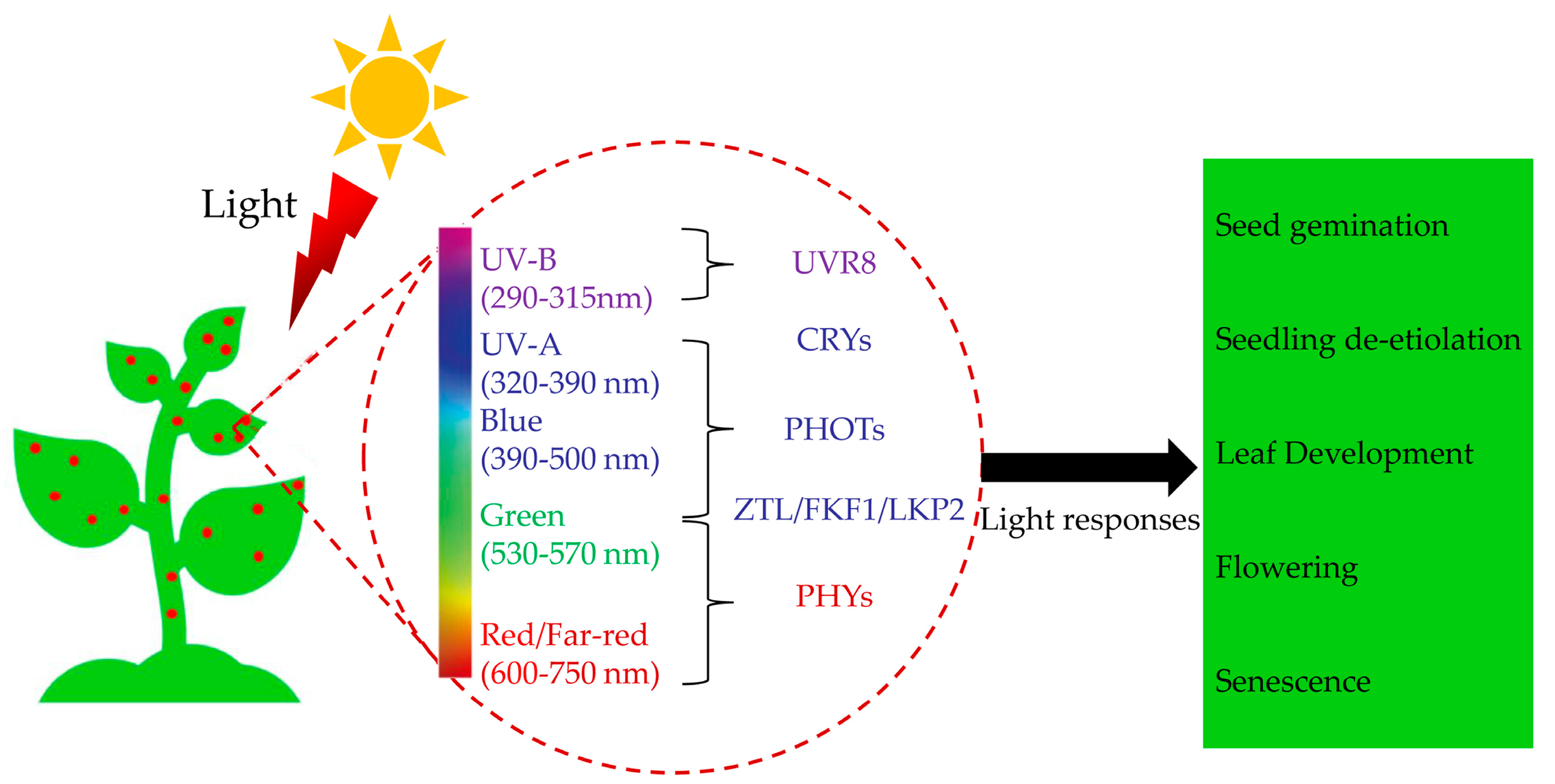This scientific diagram illustrates the process by which light, particularly UV rays, impacts a plant, detailing both absorption and subsequent physiological responses. In the top left corner, an iconic representation of the sun emits a red arrow labeled "light" pointing towards a simple lime green plant. The plant features several small red dots scattered throughout. 

Central to the diagram is a zoomed-in circular section showing a spectrum of light extending from red to UVB, represented by a gradient bar. Within this circle, different wavelengths are labeled: red, green, blue, UVA, and UVB. Adjacent to these wavelengths are brackets linking each light range to specific photoreceptors within the plant: red/far-red to PHYs, green to ZTL/FKF1/LKP2, blue to PHOTs, and UV to CRYs and UVR8. 

A black arrow labeled "light responses" extends to the right, directing attention to a lime green rectangle with categories of plant developmental stages listed from bottom to top: senescence, flowering, leaf development, seedling de-etiolation, and seed germination. This extensive labeling indicates how the plant's exposure to different light wavelengths triggers various growth and development processes.